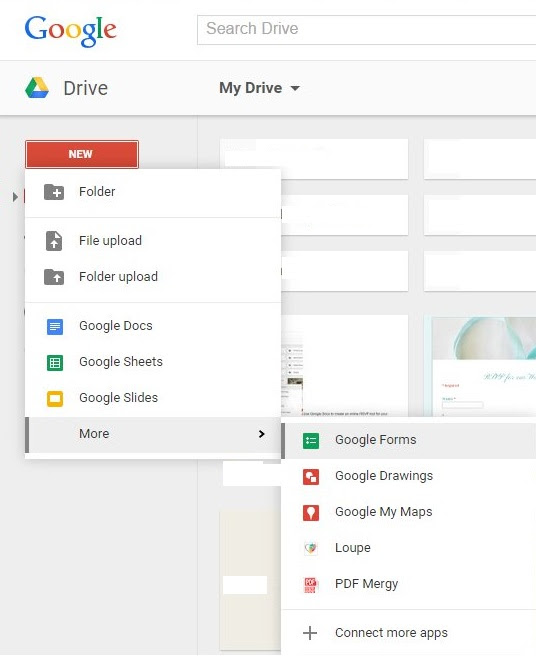The image captures a detailed view of a Google Drive webpage interface, likely on a desktop computer. On the upper left corner, the Google logo is prominently displayed in colorful letters. To the right, there are options for "Search Drive," indicating that the user is within the Google Drive environment.

Beneath the top navigation, the Google Drive icon is followed by the label "My Drive," suggesting that the user is viewing their personal drive space. There is a list of files, although specific file names are not visible. A series of options are available on the left sidebar, starting with "New," followed by "Folder," "File upload," and "Folder upload."

Further down, a suite of Google apps are listed, including Google Docs, Google Sheets, and Google Slides. An expandable "More" section, highlighted in gray with black text, reveals additional applications: Google Forms, Google Drawings, Google My Maps, Loupe (an unfamiliar term), and a PDF merging tool. Finally, there is an option labeled "Connect more apps" for integrating additional third-party applications.

Overall, the image clearly represents the Google Drive interface, detailing how users can organize, upload, and create documents and other types of files within the Google ecosystem.